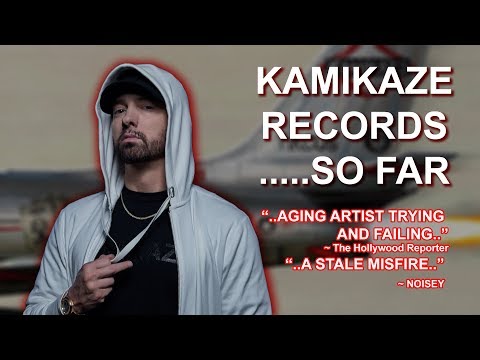This image is a promotional thumbnail for video media, potentially an advertisement or YouTube video. It features a man in his 30s to 40s, possibly of Arabic or Caucasian origin, positioned on the left side of the frame. He is wearing a white hoodie over a black baseball cap, with the hood up, a black t-shirt visible underneath, and a series of large necklaces hanging from his neck. He sports a brown goatee and stubble, and his expression is serious, almost glowering, with his chin slightly upturned as if addressing the viewer directly. His right hand, adorned with a gold watch, holds onto the strings of his hoodie.

In the background, a blurred, grey-beige silhouette of an airplane is visible, with a red and white logo on its tail, establishing an ambiguous setting. The top and bottom of the image contain narrow black strips, framing the central content. To the right of the man, large white text reads: "Kamikaze Records.... so far." Below this, outlined in red and white, are critical quotes: "Aging Artists Trying and Failing - The Hollywood Reporter" and "A Stale Misfire - Noisy." The overall atmosphere is somber, conveyed through the man's stern demeanor and the critiques displayed.